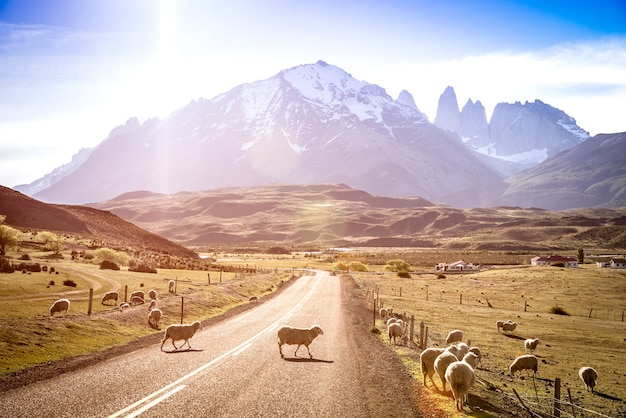A vivid daytime photograph captures a large, arid open field bisected by a two-lane road marked with a double yellow line. In the foreground, two white sheep are crossing this road from left to right, one on each side. Surrounding the road, numerous sheep are scattered across the drought-stricken pastures to the left and right. A wooden fence topped with barbed wire outlines the area, leaning slightly in the bottom right corner. The expansive landscape includes rolling hills blanketed with a mix of sparse vegetation and bare patches. In the distance, a range of jagged, snow-covered mountains rises majestically against a sky that is partly covered with wispy white clouds but predominantly blue. The sun casts a bright, late afternoon light over the scene, creating a contrast between the dry foreground and the snowy peaks in the background. Three small houses with red roofs can be seen on the right side of the image, spaced apart, adding a rustic charm to the rural setting.